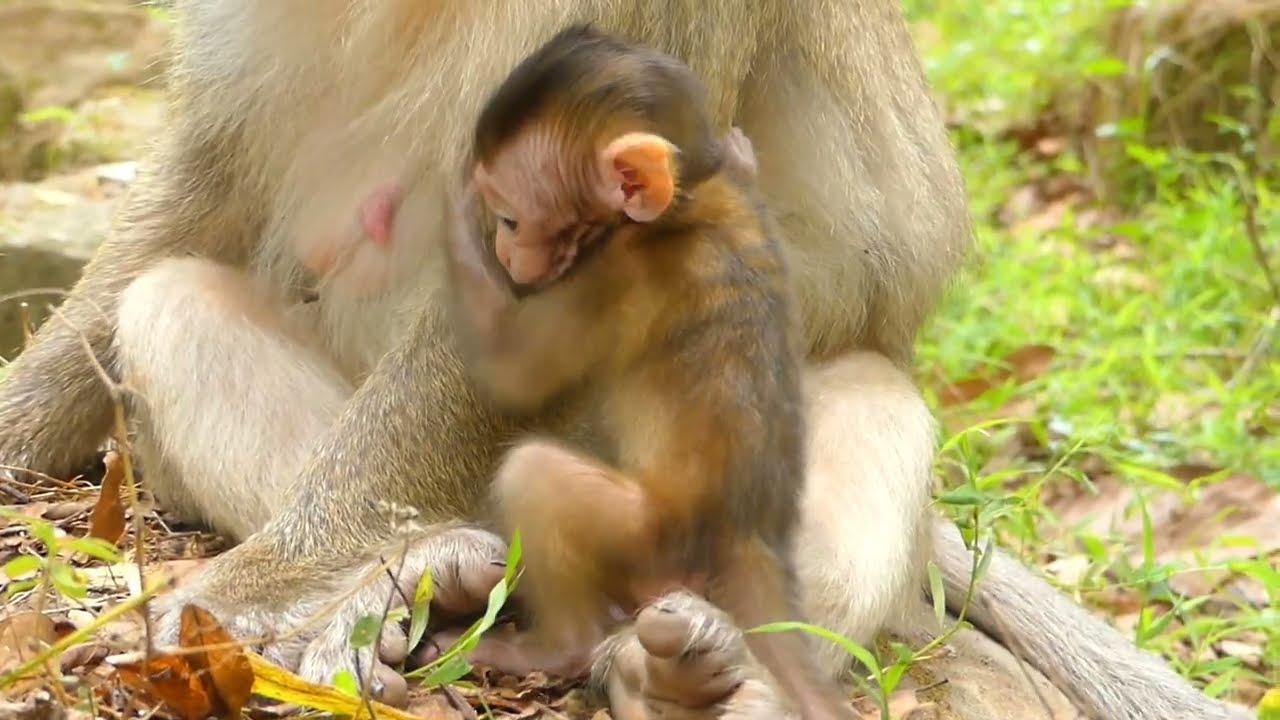This full-color, horizontally rectangular photograph captures a tender moment between a mother monkey and her baby. Taken outdoors in broad daylight, the scene unfolds on the ground surrounded by sunlit grass, scattered brown leaves, and patches of dirt. The right side of the picture is dominated by vibrant green grass and plants interspersed with light brown earth, while the left side features more brown dead leaves and rock-like surfaces. The baby monkey, with its darker brown fur tinged with orange, clings tightly to one of the mother's arms. The mother's fur is a much lighter brown, almost beige, and you can distinctly see her pink nipple as she sits, suggesting that she is actively nursing. Though the image only reveals up to the mother's shoulder, her protective posture is evident. Both monkeys' tails are visible. In the background, there are glimpses of trees, hinting at a natural habitat which could possibly be a jungle or a zoo enclosure. The sunlight illuminates not only the scenery but also highlights the delicate details of the monkeys' fur.